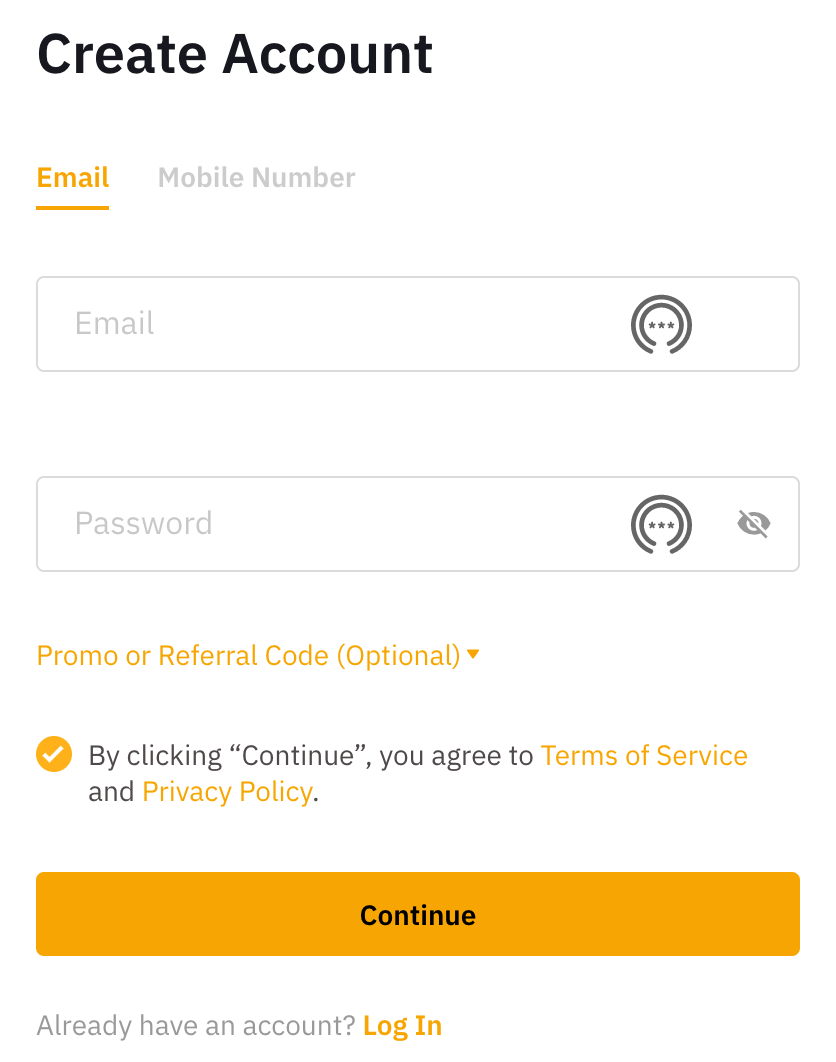This image is a screenshot of a website's account creation page. At the top, bold text reads "Create Account," with both the 'C' and 'A' capitalized. On the left side, the field label "Email" is displayed in orange text, with 'E' capitalized and an orange underline beneath it. Adjacent to it, lighter gray text reads "Mobile Number," with both 'M' and 'N' capitalized.

Below this section, there is a blank input field labeled "Email." Further down, another field is labeled "Password," followed by a space to enter a password. Beneath this field, the text "Promo or Referral Code" appears in orange, with 'P' in Promo, 'R' in Referral, and 'C' in Code all capitalized. This is followed by the word "Optional" in parentheses, with 'O' capitalized, and a drop-down arrow to the right.

Further down, there is an orange circle containing a white check mark. Accompanying this, it states, "By clicking 'Continue'," with 'Continue' in quotes, "you agree to Terms of Service and Privacy Policy." The phrases "Terms of Service" and "Privacy Policy" are in orange text.

At the bottom of the screenshot, there is an orange clickable banner with the word "Continue" in black centered text. Below this banner, the text "Already have an account? Login" is displayed, with "Login" in orange.